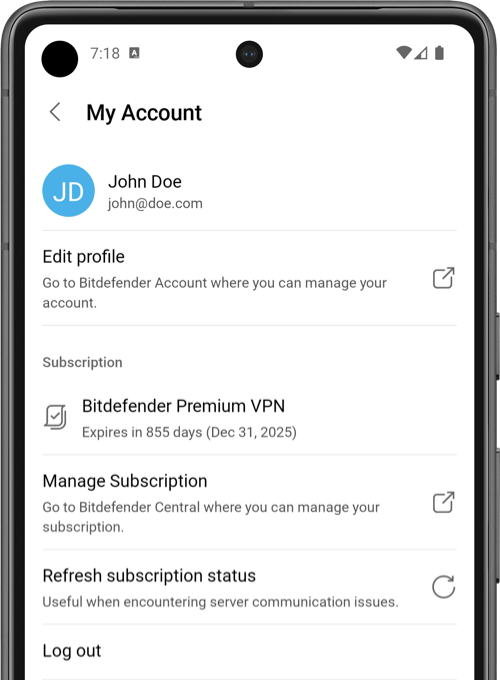This screenshot features the front face of a phone set against a white background. The phone case, which appears to be black or dark gray, frames the screen. Approximately 70% of the top portion of the screen is visible.

**Top of the Screen UI:**
- **Top Left:** A black circle icon.
- **Center:** The time displayed as 7:18 within a dark gray square icon.
- **Top Center:** Another black circle, possibly too dark to discern details.
- **Top Right:** Indicators showing Wi-Fi connectivity, cellular signal strength (two out of four bars), and a fully charged vertical battery icon.

**Main Content:**
- **Header:** Bold black letters reading "My Account," with a "less than" symbol to the left.
- **Avatar:** A blue circle with white initials "JD," representing the user "John Doe." Below the avatar, the text "John" and email "john@com" are displayed.
- **Subsection:**
  - Thin gray line
  - **Edit Profile:** Followed by "Go to Bitdefender account where you can manage your account," with an icon of a square and an arrow exiting it to the right.
- **Sub-Subsection:**
  - Thin gray line
  - **Subscription:** Bold dark gray letters. States "Bitdefender Premium VPN" with an icon of two pages and a check mark to the left. The subscription details follow: "Expires in 855 days (December 31, 2025)."
- **Manage Subscription:**
  - Thin gray line
  - **Manage Subscription:** "Go to Bitdefender Central where you can manage your subscription," with a similar square-and-arrow-exit icon to the right.
- **Refresh Subscription Status:**
  - Thin gray line
  - **Refresh Subscription Status:** Used for troubleshooting server communication issues, accompanied by a reload icon to the right.
- **Log Out:**
  - Thin gray line
  - "Log Out" is the final visible option at the bottom of the screen.

The overall layout is clean, providing clear sections for managing the user's account and subscription details.